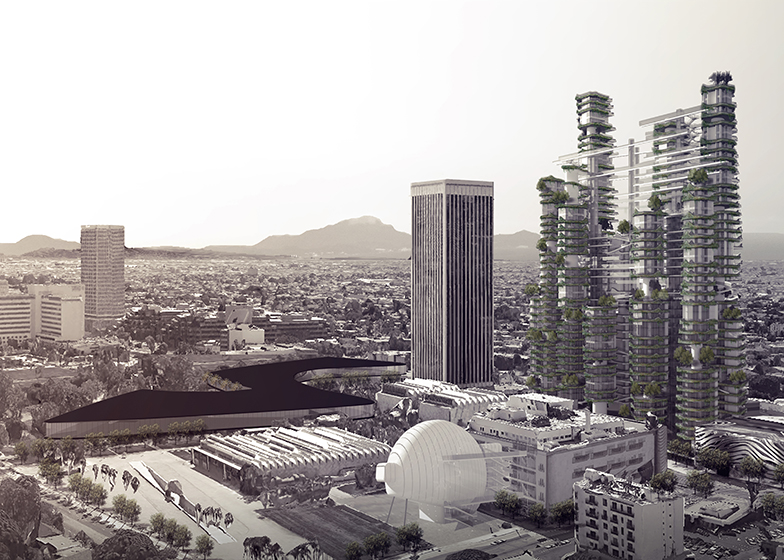This black and white photograph captures a sprawling city skyline that is wider than it is tall. The majority of the sky above the city is white, gradually shifting to a light gray on the right side. Dominating the foreground are intricate, towering skyscrapers with unique architectural designs; the tallest building, in particular, stands out with tree gardens spiraling around each level, giving it an almost futuristic appearance. Beside it, there are several other tall buildings with distinct shapes, reminiscent of a Jenga tower. Lower buildings feature rooftop gardens and streets lined with trees and parked cars, marked by their retained greenery even in the monochromatic setting. Toward the left side of the image, a long black rooftop creates a striking visual pattern, possibly appearing like a large "Z" or an "S." In the distance, the structures become smaller, leading to a horizon defined by brown mountains. This vivid cityscape exudes modernity and greenery despite its black and white palette.